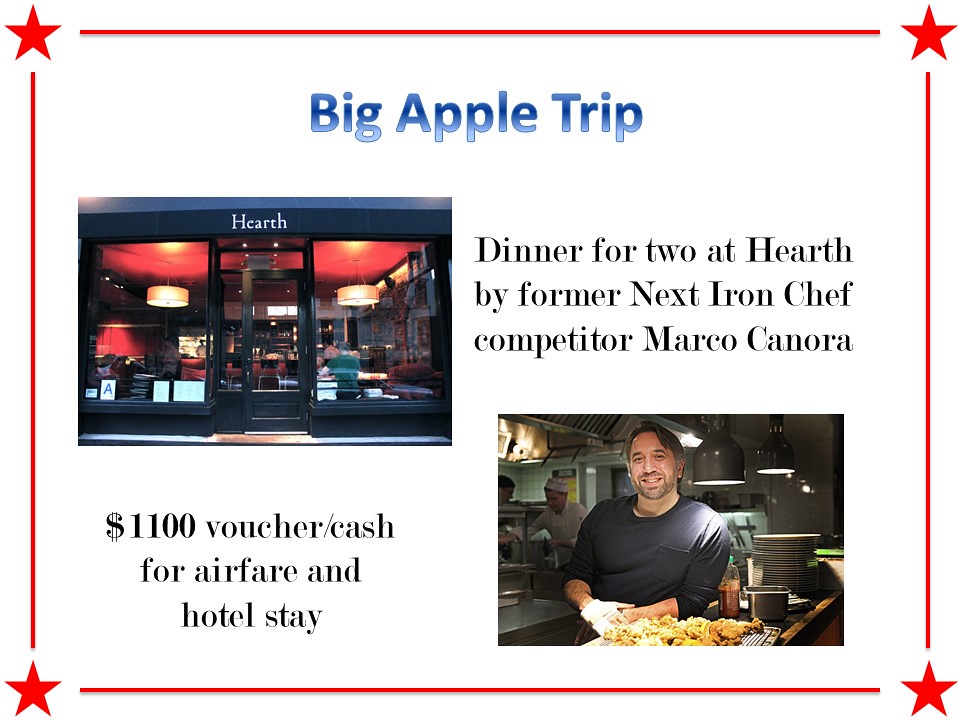The advertisement features a white background with a square, rectangular layout, bordered by red lines and a red star in each corner. At the top, bold blue letters with a gradient effect from darker to lighter blue read "Big Apple Trip." The ad includes two primary photographs: one at the upper left showing the front of a restaurant named Hearth, a black building with visible interior details like red ceilings, dim lights, and chandeliers; and another at the lower right featuring a chef in a gray shirt, smiling with short brown hair, posing inside a kitchen with food in front of him. Text within the ad highlights an enticing offer: "Dinner for Two at Hearth by former Next Iron Chef competitor Marco Canora," and also mentions a "$1,100 voucher/cash for airfare and hotel stay."